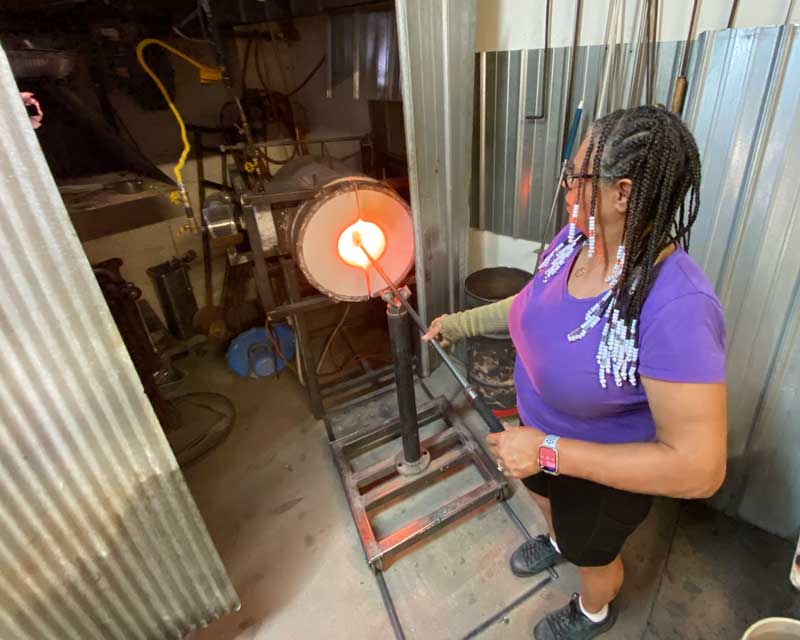In this detailed image set in a bustling workshop or factory, a sturdy and healthy black woman stands prominently on the right side. She appears engaged in welding or metallurgical work amidst an array of equipment and machinery. The environment is cluttered with various industrial items including pipes, wires, tin roofs, plastic curtains, rods, and platforms. Drums and barrels are scattered throughout the space, adding to the workshop's busy ambiance.

The woman, who has long, braided hair adorned with black and white beads, wears glasses, a short-sleeve purple top, black shorts, and black shoes. A wrist smartwatch adorns her left hand while a forearm support covers her right, aiding her as she grips a substantial metal rod. The rod she holds runs at a slight diagonal, directing towards the left where it meets a white, round hole bordered by an orange rim, suggesting it is being inserted into a hot furnace. The furnace, which sits on a metal frame, extends partially into the foreground near her feet, with the frame visibly continuing to the left side of the image.

Surrounding her are components of the workshop: silver-colored corrugated aluminum on the right side, as well as a plethora of pipes, counters, and various metal equipment that set the scene of diligent industrial labor.